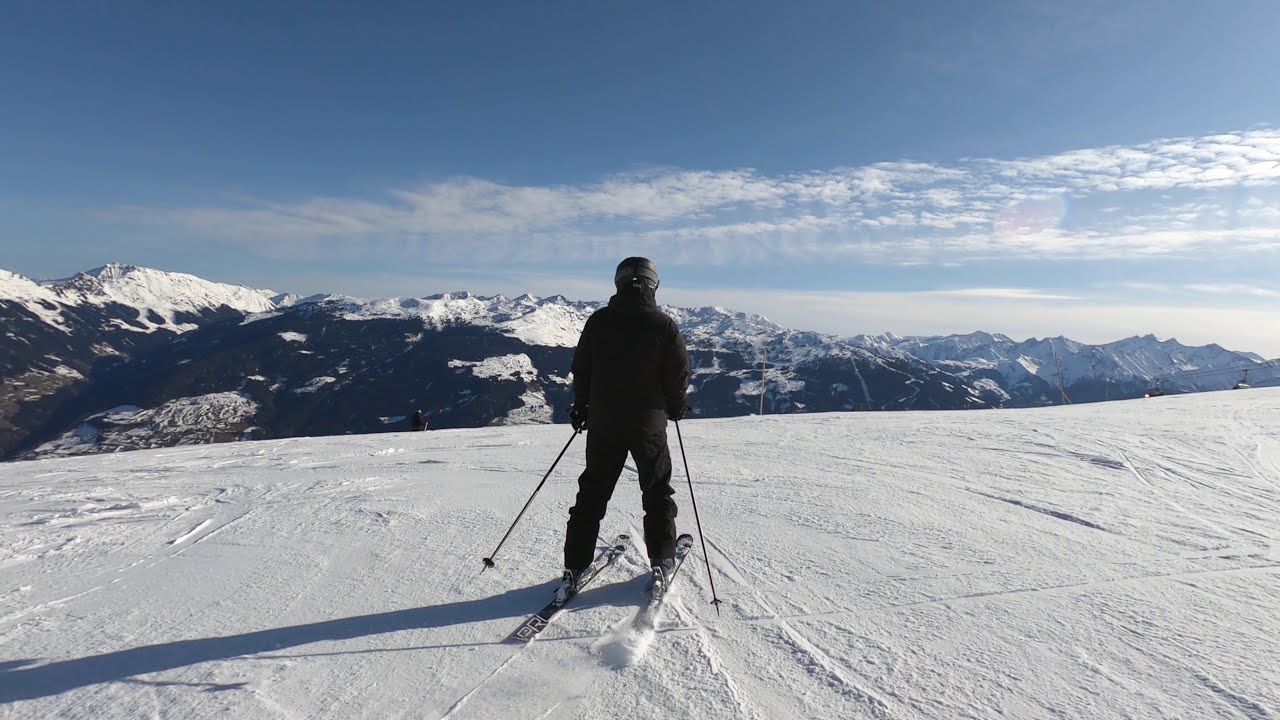This captivating daytime photograph captures a skier standing at the edge of a snow-covered plateau atop a mountain. The skier, dressed in black with a helmet, jacket, pants, and equipped with black ski poles and skis, faces away from the camera, gazing into the distance. Behind him, there is another barely visible skier on the left, near the edge of the flat, snow-covered field, which slopes slightly before dropping off sharply. The snow is packed and pristine, marked only by the tracks of previous skiers.

In the background, majestic, snow-capped mountains stretch towards the horizon, their dark slopes contrasting beautifully with the white caps and the deep blue sky above. The sky is vividly bright, adorned with long, thin, striated white clouds, suggesting high altitude. The sun casts a warm light, emphasizing the skier's shadow to the lower left. The scene is a stunning portrayal of the beauty and tranquility found in nature, with the expansive, snow-covered landscape merging seamlessly into the distant, rugged mountain ranges.